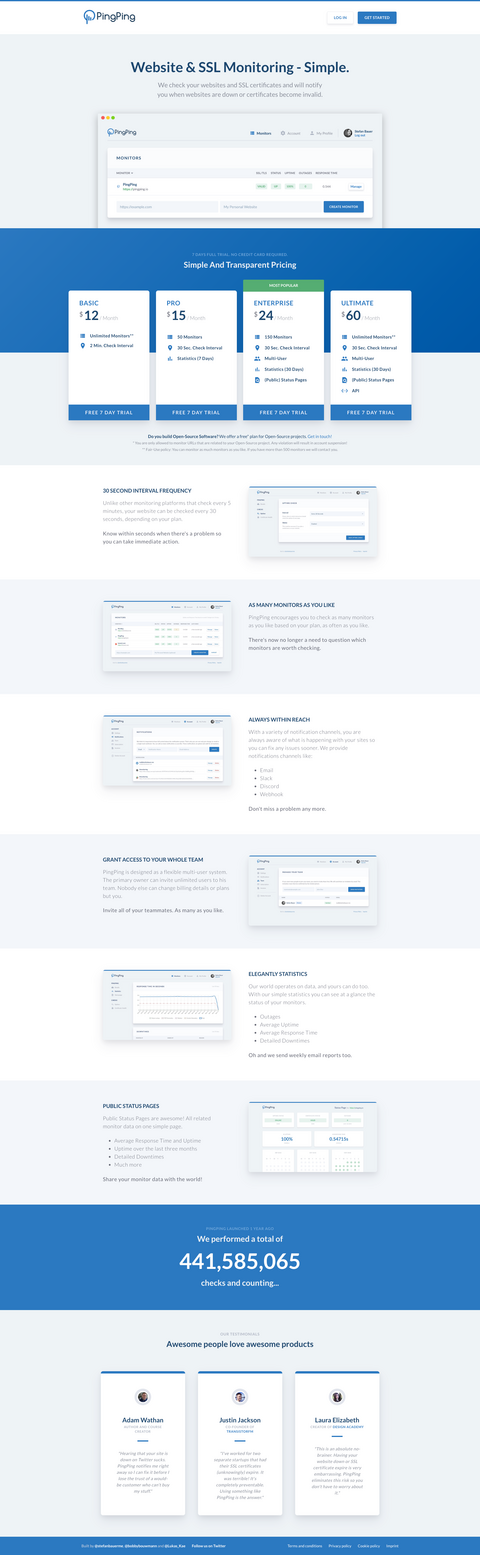This screenshot depicts a mobile-view of a website focused on website and SSL monitoring services. The image is vertically oriented and shows a series of alternating horizontal bars in shades of gray, very light gray, and white, delivering a structured, professional layout.

At the top of the webpage, there is a gray bar followed by a blue bar and another gray bar, where the text "Website and SSL Monitoring Simple" is prominently displayed along with an example screenshot. Beneath this section, a horizontal blue bar features four white squares, each with a blue footer. Each square lists a different pricing plan: $12, $15, $24, and $60, with corresponding offerings detailed under the respective prices.

Scrolling down, the layout transitions into two columns showcasing various application screenshots. The footer of the webpage is marked by a blue horizontal bar displaying a contact phone number in white text. The meticulously structured design guides the viewer from the service overview at the top to detailed pricing plans, finishing with visual application examples and contact information for further inquiries.